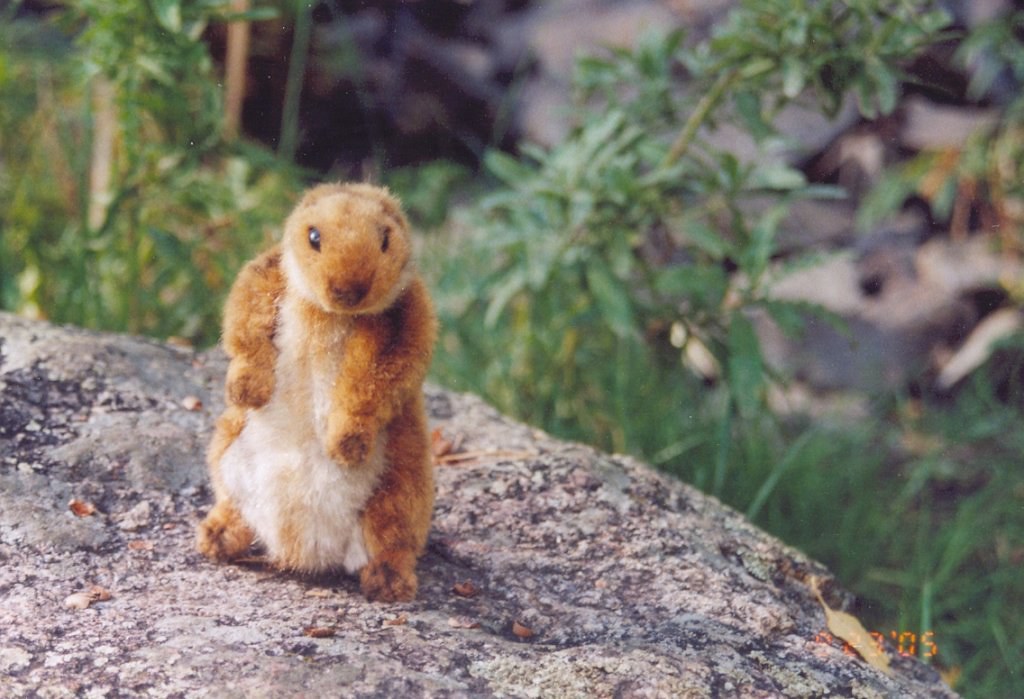The photograph is a rectangular outdoor image featuring a small, fuzzy rodent that closely resembles a chipmunk or a small prairie dog. The animal is positioned in the foreground, standing upright on its hind legs on a large, flat granite rock, with its front legs raised slightly. It has a light orangey-brown fur coat with a white or cream-colored belly. The creature has a cute, small, pointy nose and beady black eyes, which it directs straight at the camera, appearing neither afraid nor concerned. Notably, its ears are either not visible or tucked back. The background of the photo displays a blurred mix of greenery, including long grass, various plants, and possible shrubs or bamboo, suggesting a sunlit daytime setting. There is a time stamp in the bottom right corner of the image that reads “9.23.05,” marking the date the picture was taken.